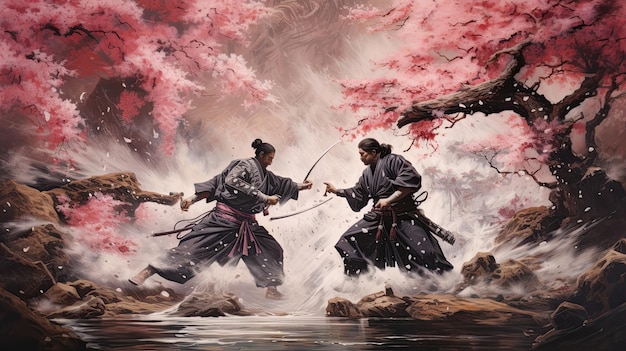The image is a highly stylized, photorealistic scene of two samurai engaged in a dramatic showdown. The background is a foggy, almost storm-like white, lending an air of mystery and intensity to the atmosphere. Flanking the scene on both the left and right are cherry blossom trees in full bloom, their branches curving inward towards the center where the samurai are clashing. They seem to be charging at each other through a river, kicking up sprays of water as they move.

Both samurai are captured in mid-action, with an almost cartoonish exaggeration to their postures. The samurai on the left, wearing a black gown cinched at the waist with a red sash, has his hair tied in a high bun. He's holding a katana in his left hand, seemingly ready for a quick draw, although the hilt of the blade is not visible, adding an uncanny quality to the image. The samurai on the right, in similar attire but with his hair in a low ponytail, strikes a peculiar stance. He holds part of a floating katana blade under his arm, with what appears to be a hilt in his hand, further emphasizing the surreal nature of the scene.

The vividness and detailed portrayal of the clash draw viewers into the moment, making them wonder what the next move will be in this tense and mysterious showdown.